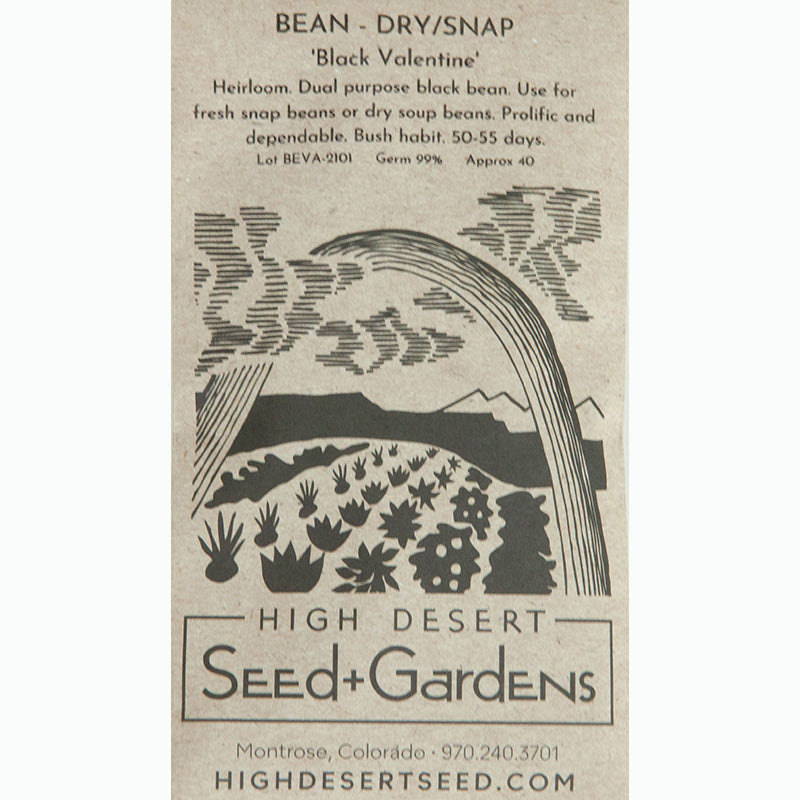The image is of a seed packet from High Desert Seed and Gardens, presented in an elegant gray, charcoal color. The detailed design at the top of the packet, rendered in a shadowed gray pencil style, introduces the product with the statement "Beans - Dry - Snap." The variety showcased is "Black Valentine," an heirloom dual-purpose black bean, suitable for both fresh snap beans and dry soup beans. The packet emphasizes the bean's prolific and dependable nature, with a bush habit maturing in 50-55 days.

The seed packet highlights key details, such as the lot number BEVA-2101, germination rate of 99%, and an approximate count of 40 seeds. A striking black-and-white illustration of a field filled with produce dominates the center. This artistic depiction includes mountains, a rainbow, and floating clouds, adding a picturesque touch to the functional item.

At the bottom, the packet provides the organization's name, High Desert Seed and Gardens, followed by the location in Montrose, Colorado. Contact details, including a phone number (970-240-3701) and the website (highdesertseed.com), are also listed, making it easy for gardeners to get in touch or learn more about the company.